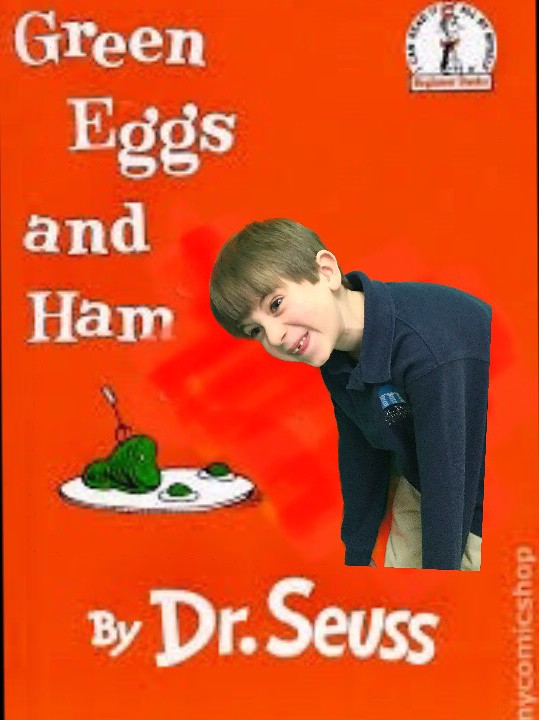This color photograph appears to be a modified version of a Dr. Seuss book cover, specifically for "Green Eggs and Ham." The background is predominantly red. In the upper left corner, white text clearly spells out the title: "Green Eggs and Ham." Directly beneath this title is the byline, also in white, reading "by Dr. Seuss." Just below the text, there is a digitally inserted image of a white plate with green eggs and ham placed on it; a fork sticks out of the ham, and the yolks of the eggs are also green.

To the right of the plate, a young boy with a bowl haircut and missing a tooth is photoshopped into the image. He is dressed in a blue top with a small logo and beige trousers, and he is smiling while looking down at the green eggs and ham. This boy is making a comical face, further adding to the playful nature of the image.

In the top right corner, there's a small circular logo featuring "The Cat in the Hat" character with some black text around its edge, indicating it's part of the Beginner Books series. Towards the bottom right corner, there is some blurry red text and a white watermark, which reads "My Commons Shop" in vertical alignment, starting from the bottom and going upwards.